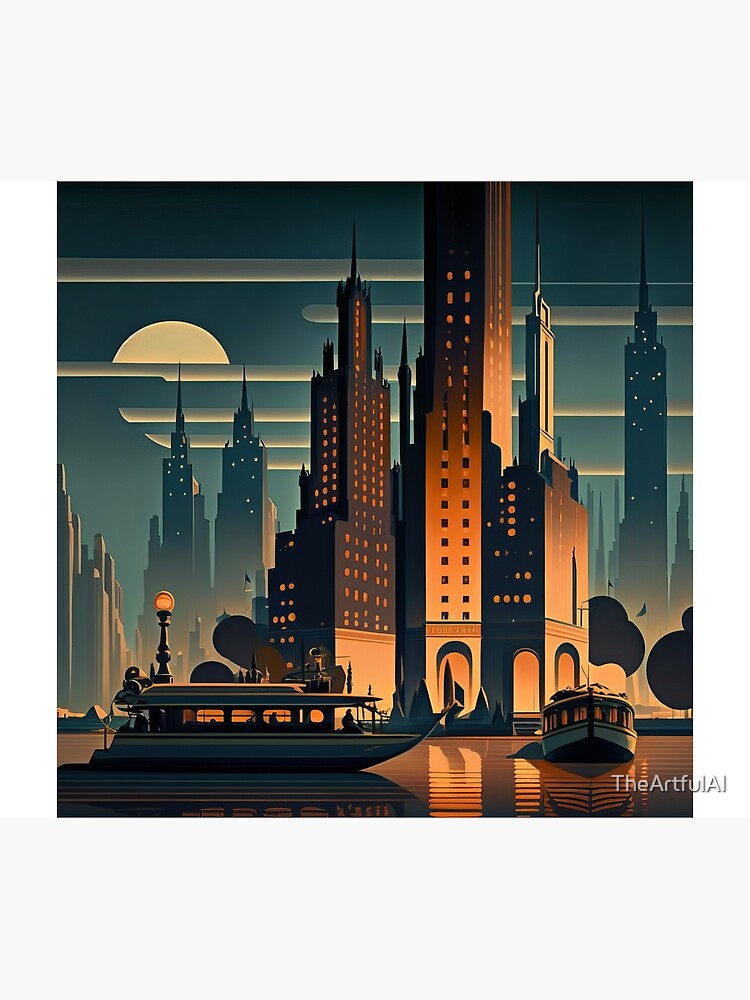This image, unmistakably AI-generated as indicated by the white text reading "The Artful AI" in the bottom right-hand corner, showcases an extraordinary cityscape. Towering skyscrapers dominate the scene, their copper-hued facades gleaming stately against the sky. These high-rise structures are adorned with numerous towers that ascend boldly, contributing to the architectural grandeur.

In the foreground, a body of water tinged with a brownish hue stretches before the buildings. Two smaller boats punctuate this aquatic expanse. One boat, with a glass-enclosed passenger area, is captured in a side view, revealing a caption at its front, suggesting motion across the water. The second boat is oriented towards the viewer, providing a clear view of its front.

Further into the distance, additional skyscrapers emerge, characterized by a bluish-gray tint. The sky above is enigmatic, featuring either the moon or the sun partially obscured by peculiar, straight-lined clouds. These elements, combined with the meticulously straight and neat lines throughout the composition, weave together a captivating urban tableau.